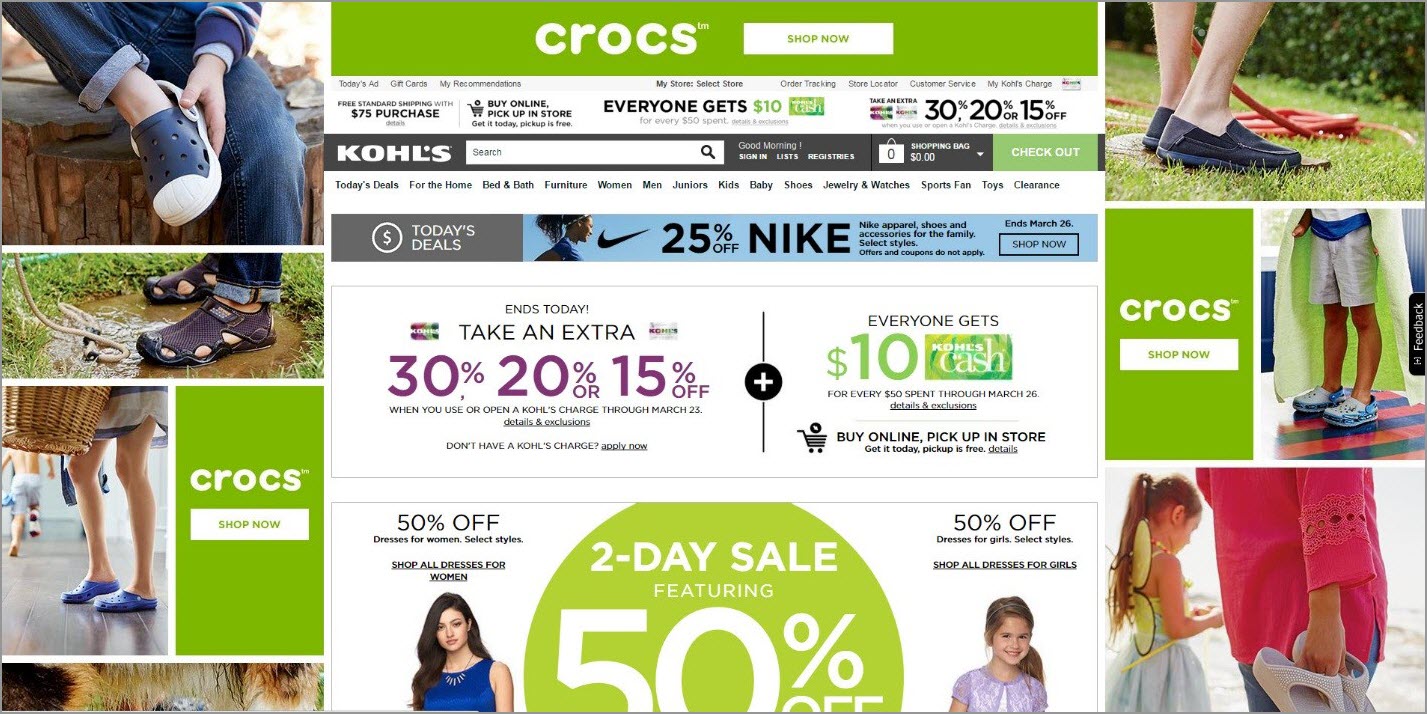The image from the Crocs website features a vibrant, promotional layout. Centered at the top is a green background with the word "Crocs" stylishly written in white. Adjacent to this, on the right, is a conspicuous white "Shop Now" button.

On the left side of the image, there's a vertical array of pictures showcasing various Crocs footwear. At the top, blue and white Crocs are prominently displayed. Just below, brown Crocs are laid out, followed by an image of someone wearing blue-colored Crocs. The green promotional background with a "Shop Now" button repeats on the left bottom side.

In the top right corner of the image, another person is pictured with black shoes in a grassy setting. Under this, yet another "Shop Now" button is featured. Further down is an image of a small child wearing gray, blue, and black shoes.

In the bottom right corner, a small girl stands on what appears to be a beach area with someone next to her holding brown shoes.

Dominating the center of the image is a prominent sale announcement. It reads: "Take an Extra 30, 20, or 15% Off. Everyone Gets $10 Kohl's Cash." Accompanying this, a banner highlights a two-day sale featuring 50% off on select items.